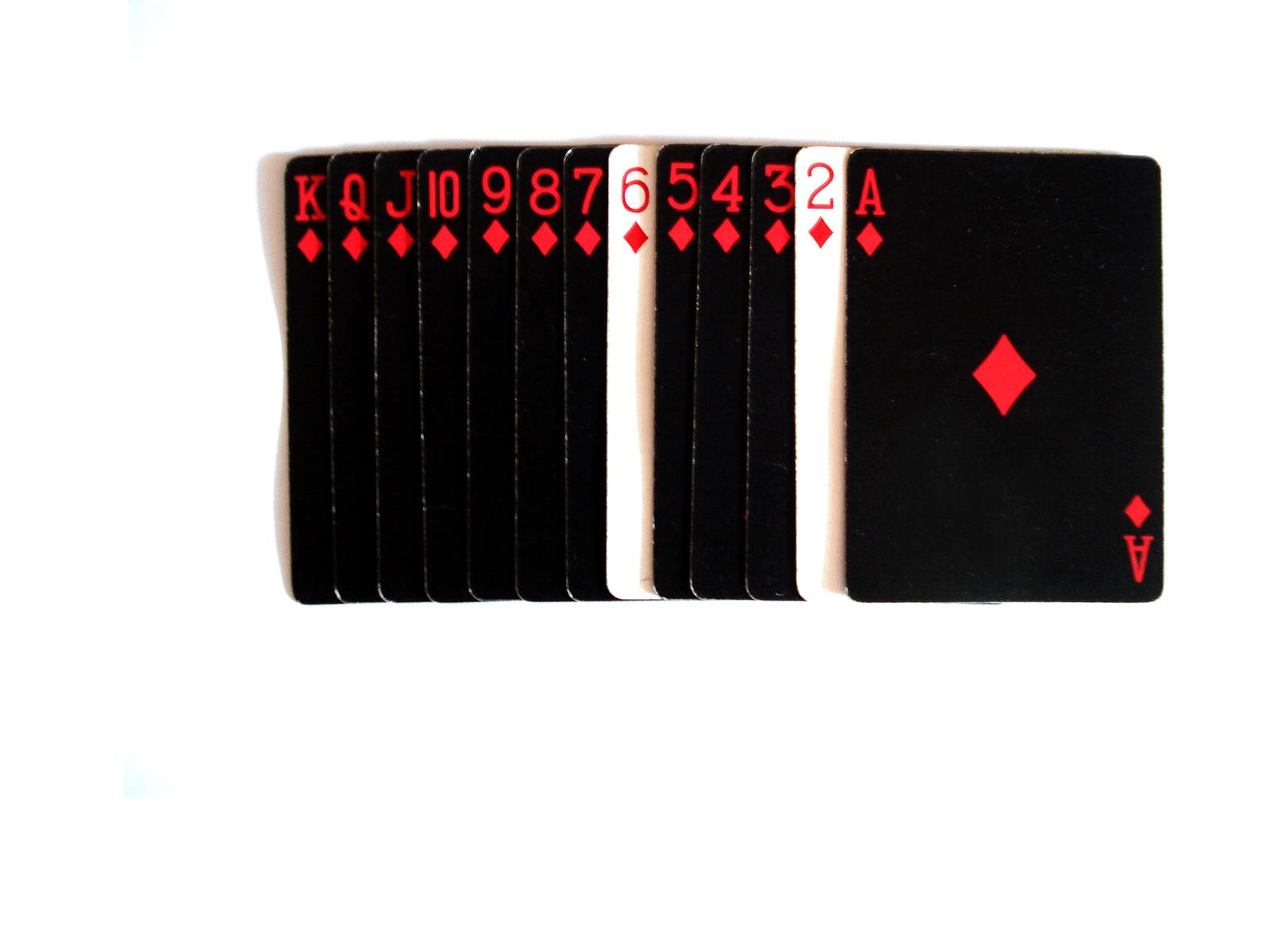The image features a partial deck of playing cards, specifically the set of diamonds, arranged neatly in ascending order from Ace to King. Most of these cards are predominantly black, with vibrant red lettering and diamond symbols, except for the 2 and 6, which are white and also adorned with red text and diamonds. The cards bear visible signs of wear along their edges, suggesting frequent use. They cast subtle shadows on the pristine, white background and on each other, adding depth to the composition. The meticulous arrangement and the contrast between the worn cards and the clean background create a striking visual narrative that emphasizes the elegance and history of the cards.